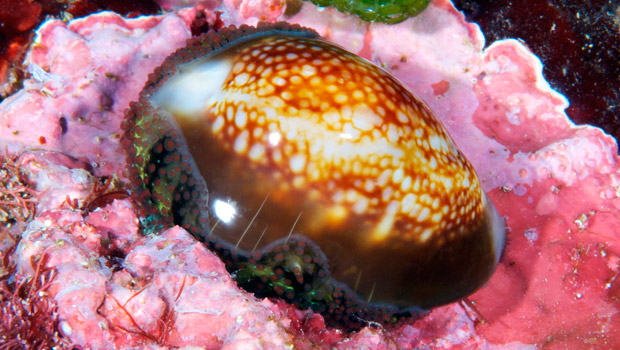The image depicts a vivid underwater scene centered around a striking coral formation. The coral, predominantly bright pink and displaying two distinct shades of pink, dominates the picture. It features a bumpy texture with some yellowish-brown areas and appears caved in at certain spots. On the left-hand side, lower corner, and the upper right corner, there are spiky protrusions, and the upper middle section includes a green glob resembling goo, with a reddish glob in the upper left corner.

In the center foreground, nestled against the coral backdrop, is an oval-shaped sea creature that resembles a snail shell. The creature displays a speckled brown pattern with a rich dark coffee brown bottom and white, irregular circular markings, reflecting light. This snail-like figure is positioned centrally, partially obscured and not clearly showing its face. 

Additionally, within the scene, the shell structure on which the creature rests has pink and white coloration, possibly depicting an artistic interpretation of a sea creature with an opaque white body and orange internal accents. The surrounding elements, including green and red tentacle-like formations, contribute to the intricate and colorful marine environment captured in this detailed photograph or artistic representation.